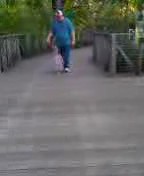In this slightly blurry, small-scale photograph, an adult male, who could either be a father or an uncle, is seen walking hand-in-hand with a young child along a boardwalk in a park. The man is dressed casually in a blue t-shirt, jeans, and a white baseball cap. The child, whose details are harder to discern due to the image quality, appears to be wearing light-colored clothing that seems to be a blend of whitish and pinkish hues. The wooden slats of the boardwalk are clearly visible, creating a defined path bordered by railings on both sides. Beyond the boardwalk, lush greenery, likely consisting of shrubs and trees, offers a natural backdrop to this serene moment. The overall blurriness and small size of the picture obscure finer details, but the essence of a tranquil walk in a park setting is captured.